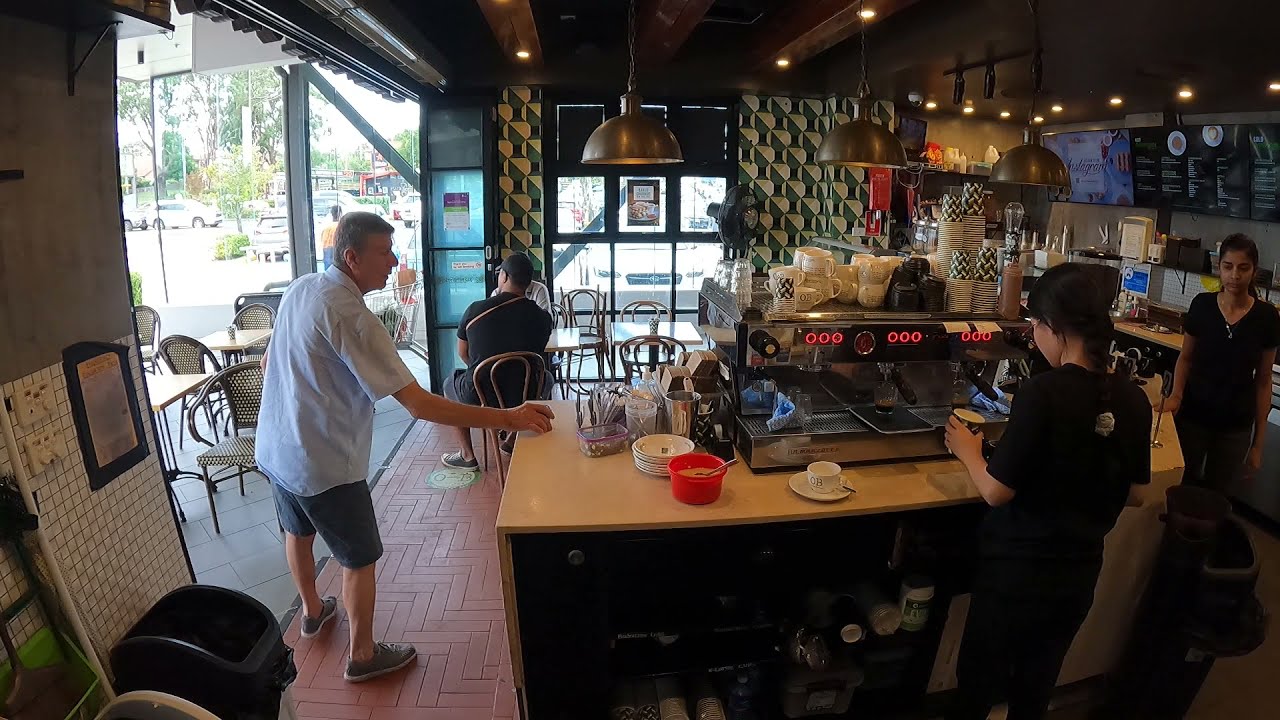In this highly detailed photograph taken from behind the counter of a cozy, bustling coffee shop, the intricate setup of the coffee machine and various utensils on the light brown wooden countertop is clearly visible. Cups of different sizes, bowls, condiments, and napkins are neatly arranged on the counter, with a drink-dispensing tap situated to the right. 

A barista, with light brown skin, her black hair braided and pulled back, is diligently preparing coffee. She is dressed in a short-sleeved black shirt and black pants, working skillfully with the equipment. On the side of the counter, a Caucasian man in a white shirt and gray shorts reaches out to grab some napkins, his right hand touching the counter. 

The interior of the coffee shop features green and white wallpaper and decorative hanging lights from the ceiling, creating a warm and inviting atmosphere. Additional countertops in the background house a menu and what looks like a dishwashing station. To the left, there's an open space with a pull-down metal closure. 

Beyond the window and door, the outside daylight filters in, highlighting tables and chairs dotting the exterior space, with a road and several vehicles visible, suggesting a lively street just outside the tranquil, welcoming coffee shop ambiance.